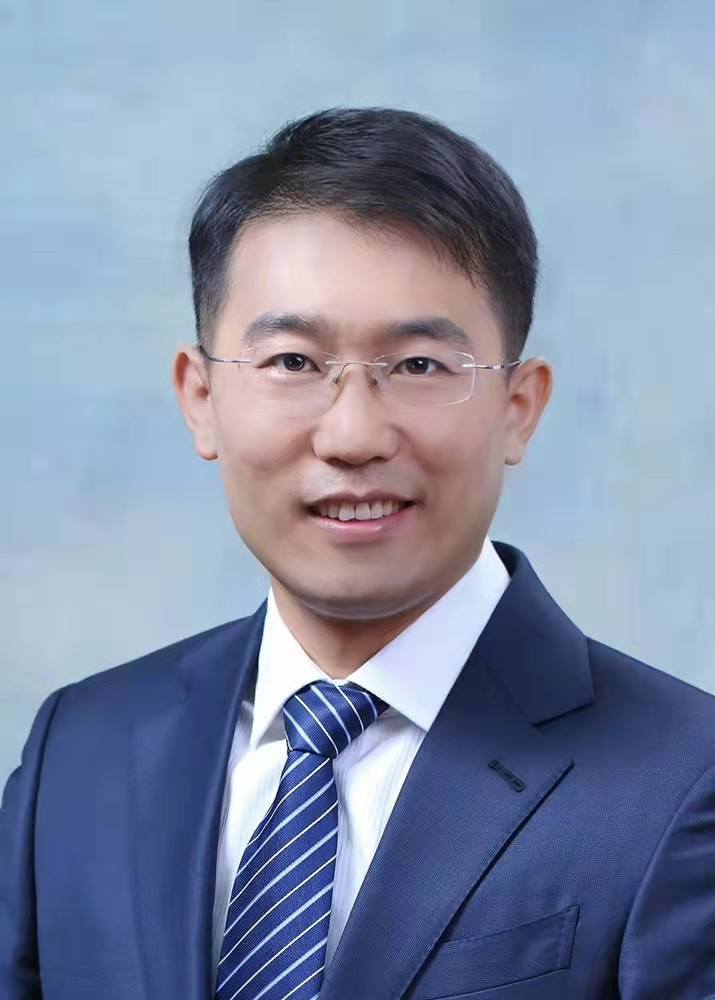This is a detailed portrait of a young Asian man in his 20s or 30s, captured against a pale, textured light blue background. He has neatly combed dark hair, parted to the side with a swoop across his forehead, and the sides of his head feature a fade-style haircut. His facial features include slightly bushy eyebrows, brown eyes, a flat nose, very high cheekbones, and an elongated face. He is grinning broadly, showing his top row of teeth, with a slightly elongated front tooth on his left side. The man is wearing a navy blue suit jacket, a white button-up shirt, and a blue tie with baby blue and yellow stripes. His glasses are relatively small, oval-shaped, and frameless with thin silver side frames and a silver bridge. There is a button hole on the collar of his suit coat, and his tie is tightly knotted. He exudes a warm, confident demeanor as he smiles toward the left side of the image from the viewer's perspective.